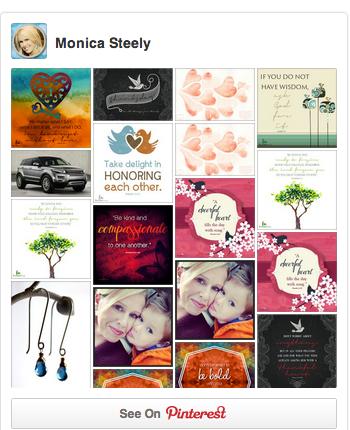This image is a detailed screenshot from a Pinterest page, showcasing the account of Monica Steele. The background is a white rectangle, and in the upper left, there is a small, slightly tilted photograph of a smiling woman with blonde hair and black eyebrows. Her name, "Monica Steele," is written in black text next to the image. Below this is a grid of various images and advertisements arranged in four columns.

In the first square directly under Monica Steele, there is a landscape picture transitioning from a blue background at the top to brown at the bottom, with a dark brown heart in the center. Next to it is a dark black square featuring a ribbon with black lettering and a white image on top. Adjacent are two identical images of hearts in shades of pink, one above the other.

Further down, in the center of the grid, there are two photographs of the same woman, presumably Monica, with a child, their cheeks touching. Below the heart image, there is a picture of a silver vehicle, and next to it, an image of a green tree with an overlaid text. Below the tree image, there's a branch adorned with blue teardrop crystal earrings.

In the second column over, second row down, there is an image with two birds and the text "Taking Delight, honoring each other." Underneath this, a dark red background with orange text is visible, though the specific text is unreadable. On the third row of the third column, a pink background with a white circle in the center displays the text "Dearest Friend."

At the far right corner of the grid, the uppermost image bears the text "If You Do Not Have Wisdom," followed by unreadable handwritten words. The bottom right image features white writing on a black background with a small black item on top with indistinct points. At the very bottom of the page, a gray rectangle banner contains the phrase "See on Pinterest" with "Pinterest" highlighted in its distinctive red script.